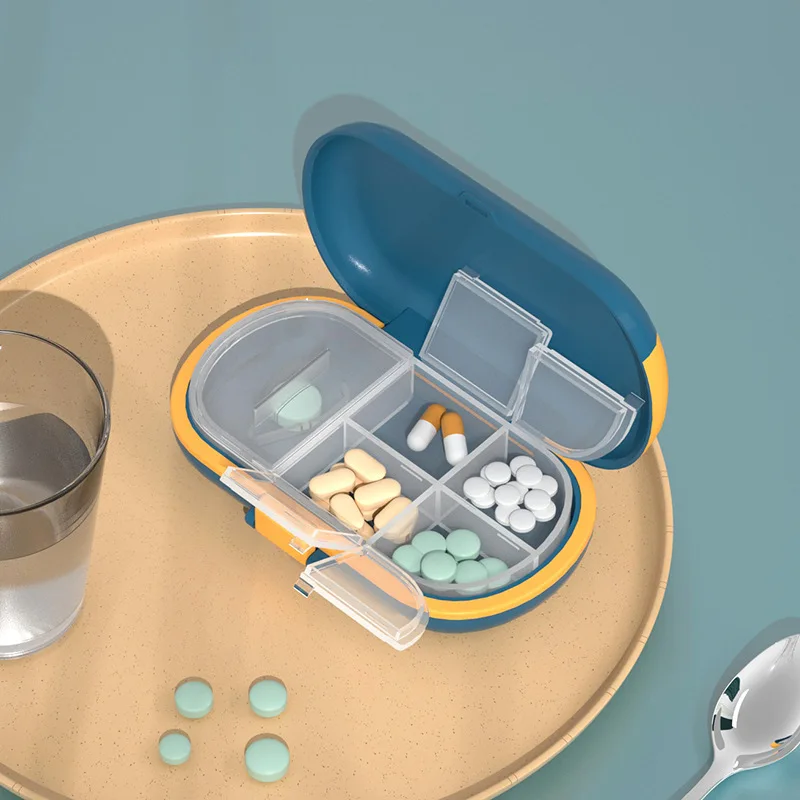The illustrated image vividly depicts a setup of a pill management system on a peach-colored plate with darker brown speckles, resembling a hospital plate. Central to the composition is an oval-shaped pill case, primarily light blue with yellow outlining, and featuring a translucent, opaque lid lifted upright. This case has five compartments, four of which are open, revealing a variety of pills. 

In the top left compartment, tan and white capsules are visible, while the compartment to the right contains small white circular pills. The lower right compartment houses teal-colored circular pills, and the bottom left compartment has peach-colored oval capsules. Positioned on the left side of the plate is a partially visible glass tumbler filled with water. Adding to the detailed setting, a silver spoon rests at the bottom right of the plate. The background of the entire scene is a light blue color, complementing the detailed elements of the image.